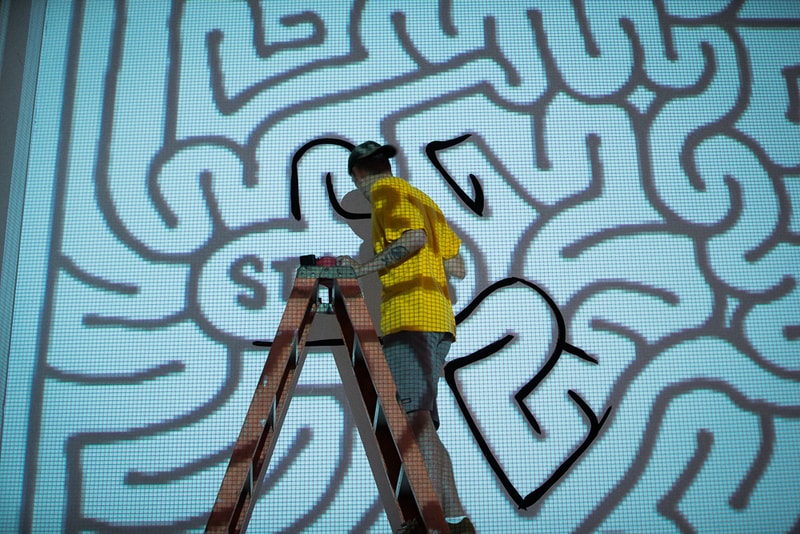In the image, a man is painting a large mural that is being projected onto a white wall. He is standing a few rungs from the top of an orange ladder, with his left hand touching the top for balance. Clad in a yellow T-shirt, gray shorts, dark shoes, and white socks, he also sports a backwards dark ball cap and a tattoo on one arm. The mural design resembles a black-and-white maze with organic, brain-like curves, and he is currently working near a section marked "start." The projector illuminates both the wall and the man with small grid lines, casting soft shadows that add depth to the scene. Although he is early in the process and hasn't made much progress, he is meticulously tracing the projected pattern with precision.